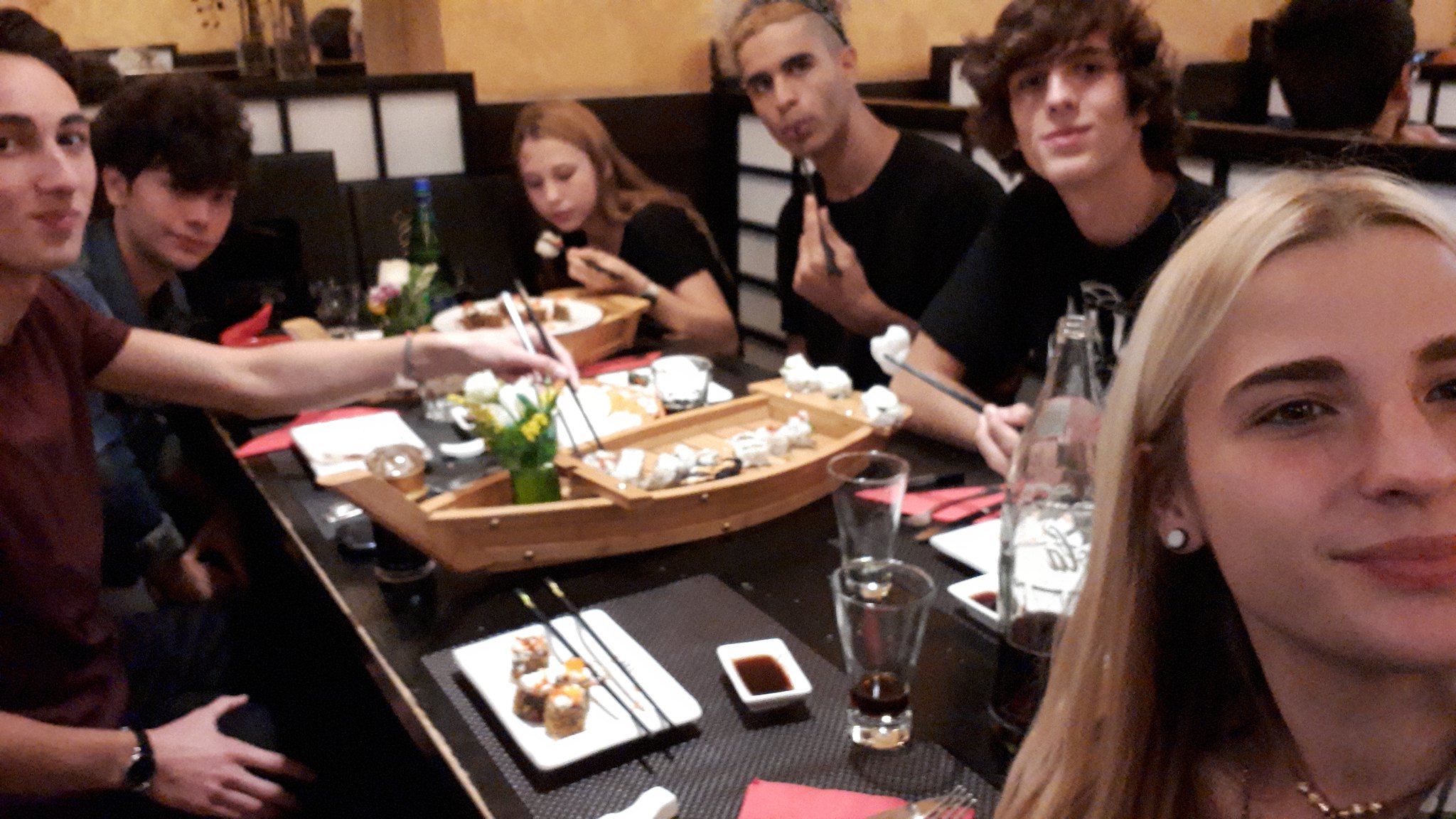In the image, there is a group of six young adults, likely teenagers or college-age, gathered in a spacious restaurant booth for a dinner outing. They appear to be enjoying a sushi meal, which is prominently served on a wooden sushi boat placed in the middle of the brown table. The sushi boat, adorned with flowers at the front, is surrounded by white plates, chopsticks, soy sauce in white containers, and an assortment of drinks including glasses and a bottle, possibly containing soda or wine. 

The group consists of four boys and two girls, most of whom have dark brown hair while two have lighter orange-light brown hair. They all exhibit beige-peach skin tones typical of European descent. They seem to be preparing to take a group selfie, as everyone is looking towards the camera with subtle smiles; however, one girl continues to eat, and one boy has a chopstick in his mouth while still engaging with the camera. 

The ambiance of the restaurant is characterized by tan or gold-colored walls and white lights. Other customers are faintly visible in the background, reinforcing the setting as a busy dining establishment. The table is equipped with rubbery placemats, complementing the overall aesthetic of the dining experience.